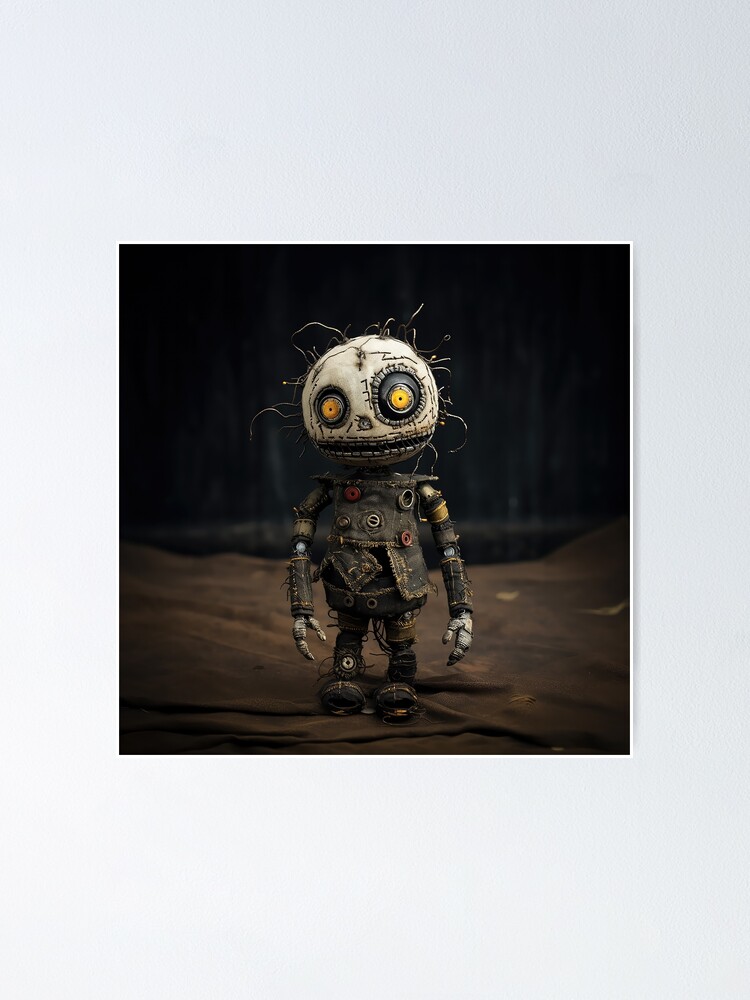The image depicts a Tim Burton-esque, humanoid doll or sculpture standing upright against a predominantly black background. The figure's round, white head features large, circular eyes with yellow irises and tiny black pupils, a button nose, and a mouth that appears partially sewn shut. Wisps of scraggly wire serve as its hair. The figure's body is a patchwork of various fabrics, adorned with buttons and metal trinkets, wearing a tattered leather jacket and pants. It stands atop old, dusty, wrinkled brown fabric. The overall aesthetic evokes a style reminiscent of the "Nightmare Before Christmas" movie, with distinct elements of stitchwork and a whimsical, eerie vibe. The background is bordered by light gray, framing the character that brings an animated, cartoon-like quality to the image.